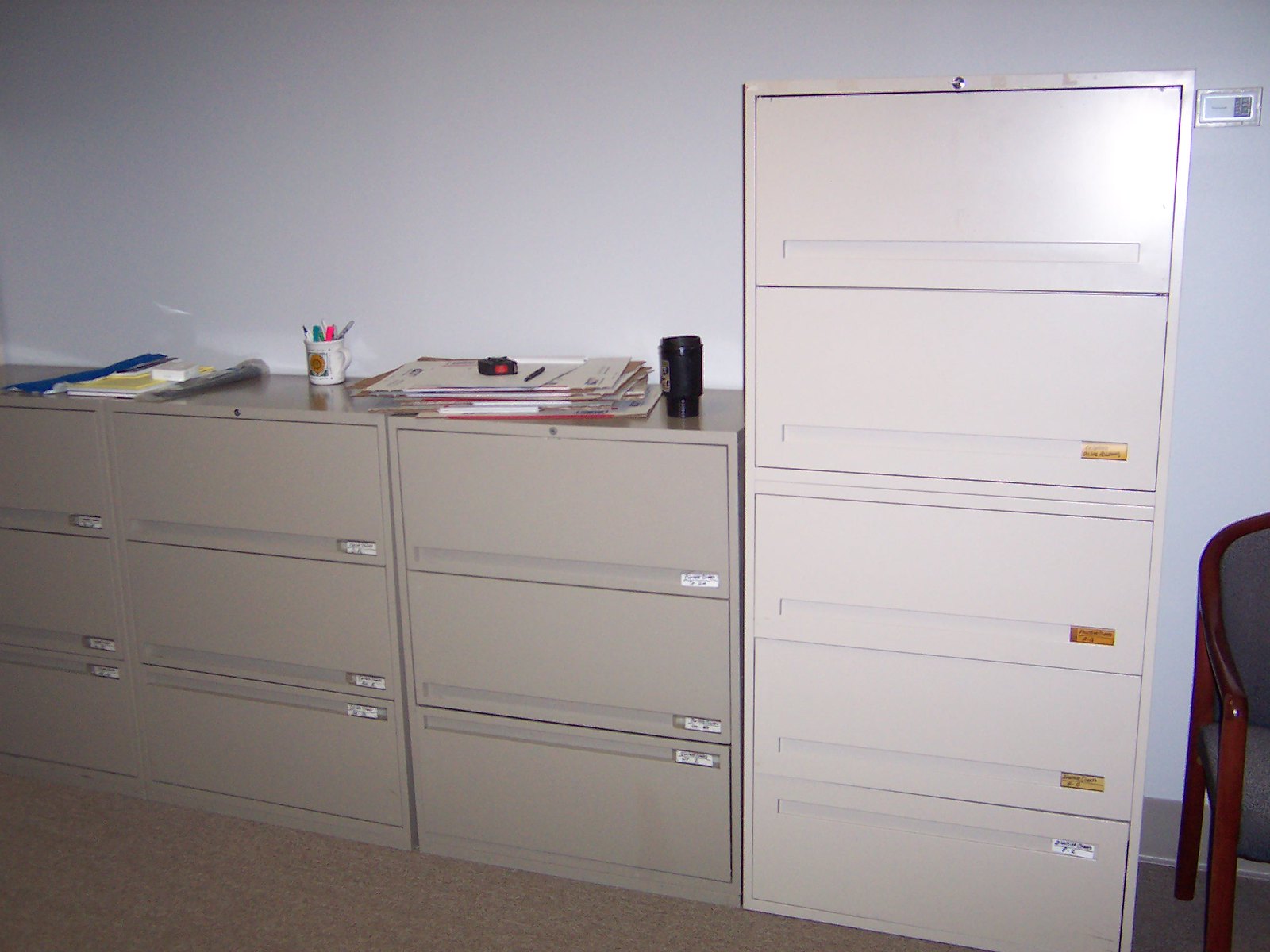The image captures a section of an office room with distinct filing cabinets and various office supplies. On the left side, there are three shorter filing cabinets, each with three drawers in a brownish or grayish hue, while on the right, there is a taller, cream-colored cabinet with five drawers. The cabinets are topped with several items: a cup holding pencils and pens, stacks of papers featuring yellow, white, blue, and gray lines, and a pile of clipboards with a small black rectangle featuring a red dot on top. Additionally, there is a black portable water cup. A wooden chair with gray, padded cushions is positioned on the far right near the bottom. The room is lit with natural daylight, though the lighting appears somewhat subdued. The walls are painted in varying shades of gray, shifting from a darker gray on the upper left to a lighter gray on the right. A darker gray strip is present along the lower part of the wall. Brown carpeting covers the floor, and the overall atmosphere suggests a utilitarian office setting.